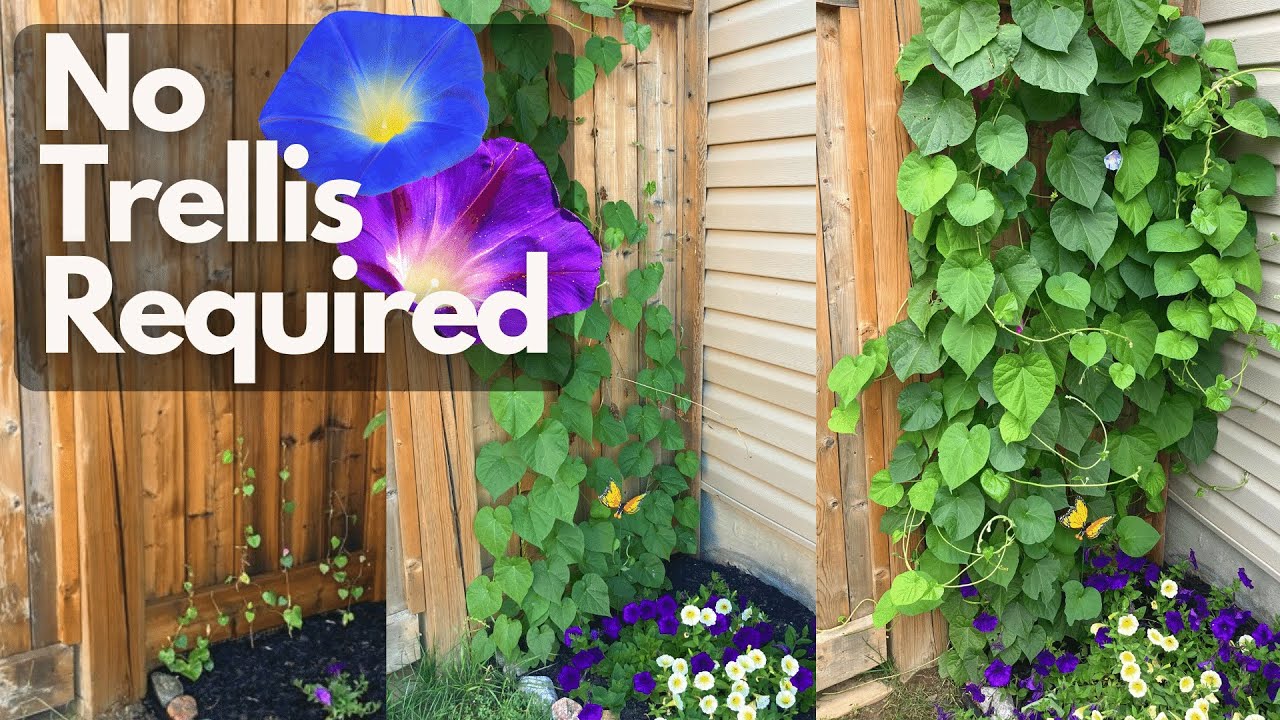The image showcases the transformation of a wooden fence through three stages of vine growth, emphasizing the progress with a caption in a white, sans-serif font that reads "No Trellis Required" against a light gray, transparent text box. In the first stage, only a few ivy leaves are sprouting from the ground amidst black dirt, starting their journey up the brown wooden fence. The second stage displays more extensive vine growth, now partially covering the fence and accompanied by bright royal blue and purple flowers at the bottom. The final stage reveals a lush, fully-grown ivy that envelops the entire wooden fence and even encroaches on the siding of a nearby structure, with purple and white flowers still visible at the base. The phrase "No Trellis Required," highlighted by a black faded background with two colorful flowers, underscores the robust, self-sustaining nature of the vines.